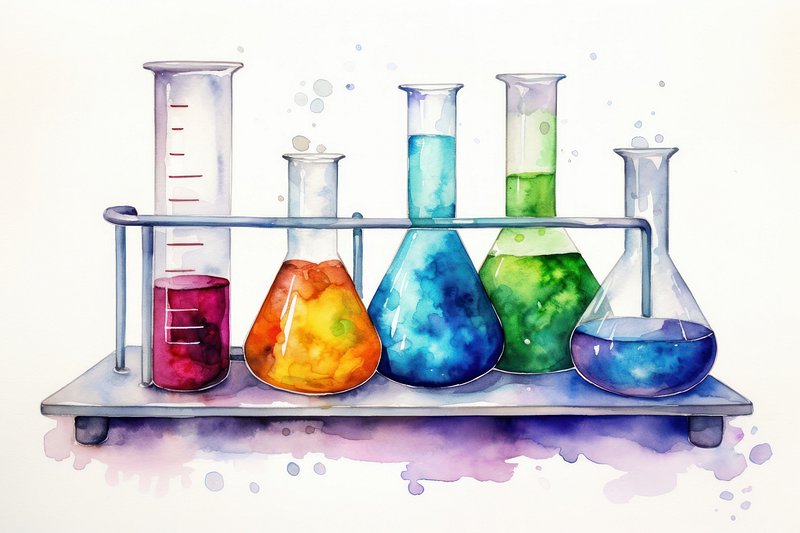This is an intricately drawn illustration resembling a chemistry lab setup, featuring five glass beakers of varying shapes and sizes, neatly arranged on a small, metallic stand. The transparent beakers contain an array of vividly colored liquids, each with distinct characteristics and bubbling textures.

The first beaker, tall and slender with measurement lines, holds a reddish liquid that reaches up to the third mark, while the bottom remains filled with a pinkish hue. Next to it, a shorter container with a rounded, triangular bottom contains a dynamic mixture of orange and yellow, bubbling vibrantly.

The third beaker showcases a captivating blend of blue and green, almost filled to the brim. Moving on, the fourth beaker is about halfway filled with various shades of green, including patches of darker and lighter green, interspersed with pinkish tinges and bubbles.

The final beaker stands shorter, holding a modest amount of blue liquid mixed with purple, bubbling slightly. Underneath the entire setup, splashes of pink and accents of purple and blue enhance the artistic background, adding a touch of whimsy to the scientific depiction.